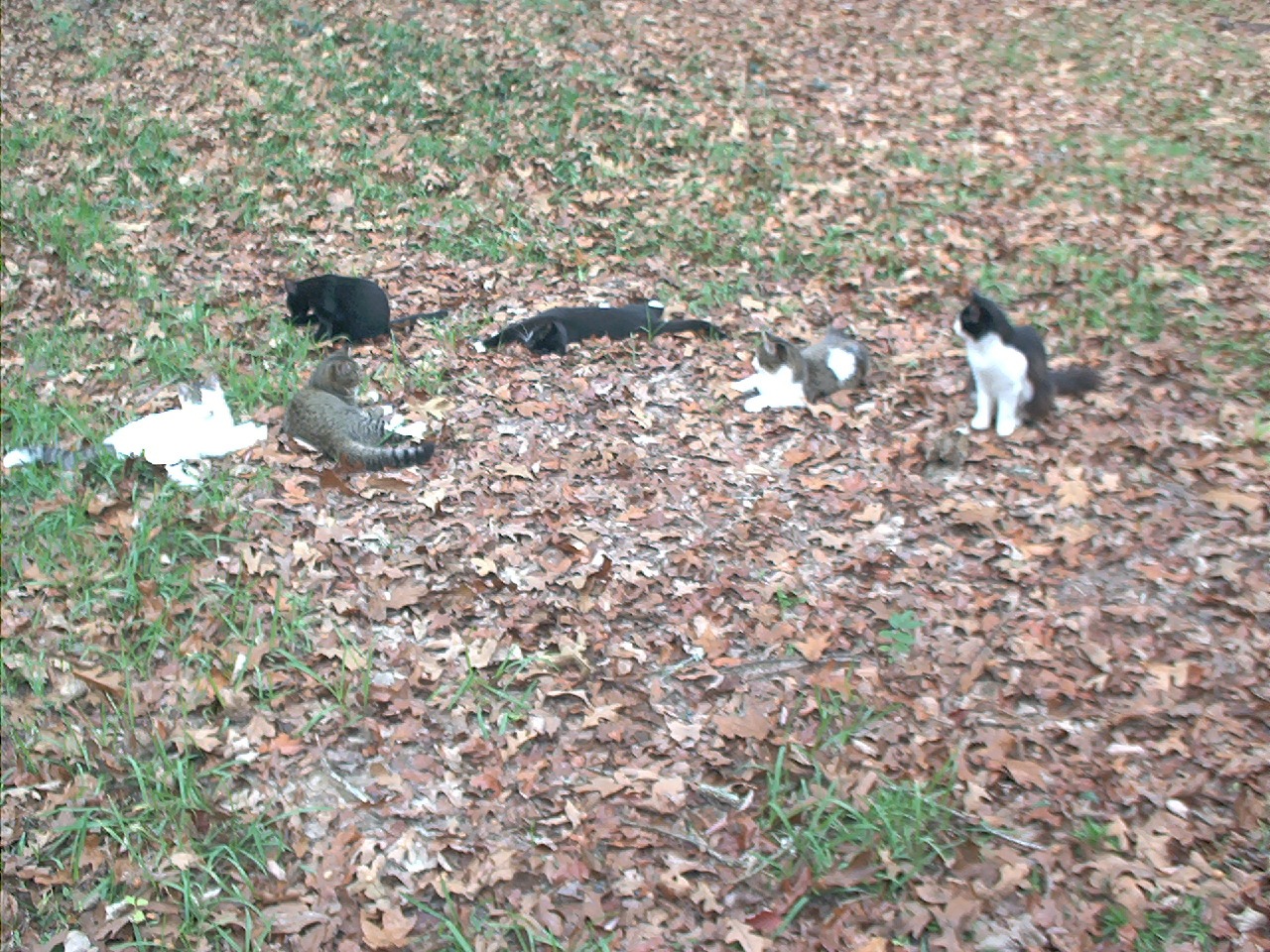In the image, a seemingly serene, leaf-strewn field encompasses a collection of six cats, creating a bucolic tableau. The earth is lightly blanketed with brown and orange fallen leaves, among which sparse blades of grass peek through. At the central point of the picture, slightly offset to the left, sits a stark white trash bag, subtly contrasting the natural earthy tones.

Starting from the right, we observe a black and white cat; it sits upright with a black back and a harmonious white underbelly, neck, and paws. Just to the left, a gray cat turns its head to the right, displaying a predominantly gray body with a white spot on its back. This cat’s tail is gray, tipped with black. Adjacent to this, a fully black cat appears to be grooming itself, its head lifted as if mid-lick.

Continuing leftward, another black cat lies stretched out languidly on its side, its black fur occasionally interrupted by white paws. Below and to the left of this cat is a tabby with brown and white fur – it sprawls flat on its stomach, showing a brown back and head, contrasting with its white chest and legs. Furthest left, a white cat with a gray tail completes the scene, lying down peacefully.

This assembly of cats in their various poses and colors creates a harmonious blend with the autumn landscape, each cat seemingly oblivious to the photographic observer.